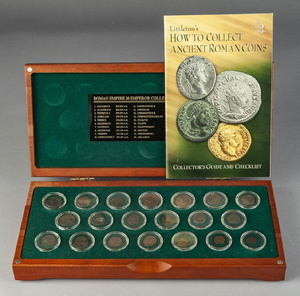This photograph showcases an impressive collection of ancient Roman coins, meticulously arranged within a sophisticated wooden display box. The box, crafted from rich brown wood, is elegantly lined with a lush green velveteen surface, providing a regal backdrop for the historical treasures it holds. The box is open, revealing its contents, and a small pamphlet titled "How to Collect Ancient Roman Coins" is propped upright against the inner lid, indicating the thematic focus of the collection. The coins are securely placed in three distinct rows of specialized impressions, with the top and bottom rows each containing seven coins, and the middle row housing six coins, highlighting the careful organization and presentation of this striking assemblage.